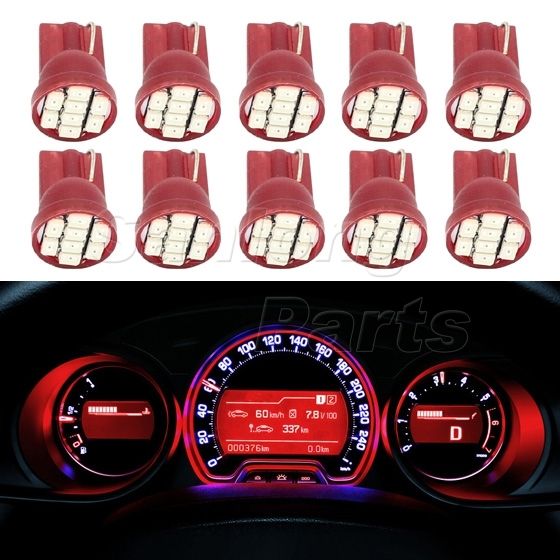The advertisement showcases two main images. The top half features an array of 10 identical red, bell-shaped LEDs, each containing 8 white rectangles with central dots, arranged in groups: 2 rows of 5, with configurations of twos and a central column of four. Beneath this, the bottom half of the advertisement displays a car's illuminated dashboard focused on three large circular dials. The central dial indicates the speedometer in kilometers per hour, currently showing 60, with an arrow pointing to 60 and the odometer reading slightly over 3,000 RPMs. The fuel gauge shows the tank is half full, and a digital display reads 337 kilometers, suggesting the car is possibly new. The entire dash is lit in a red and white scheme with some purple hues, and there's a partially visible watermark reading “parts” overlapping a heart shape on the upper right.